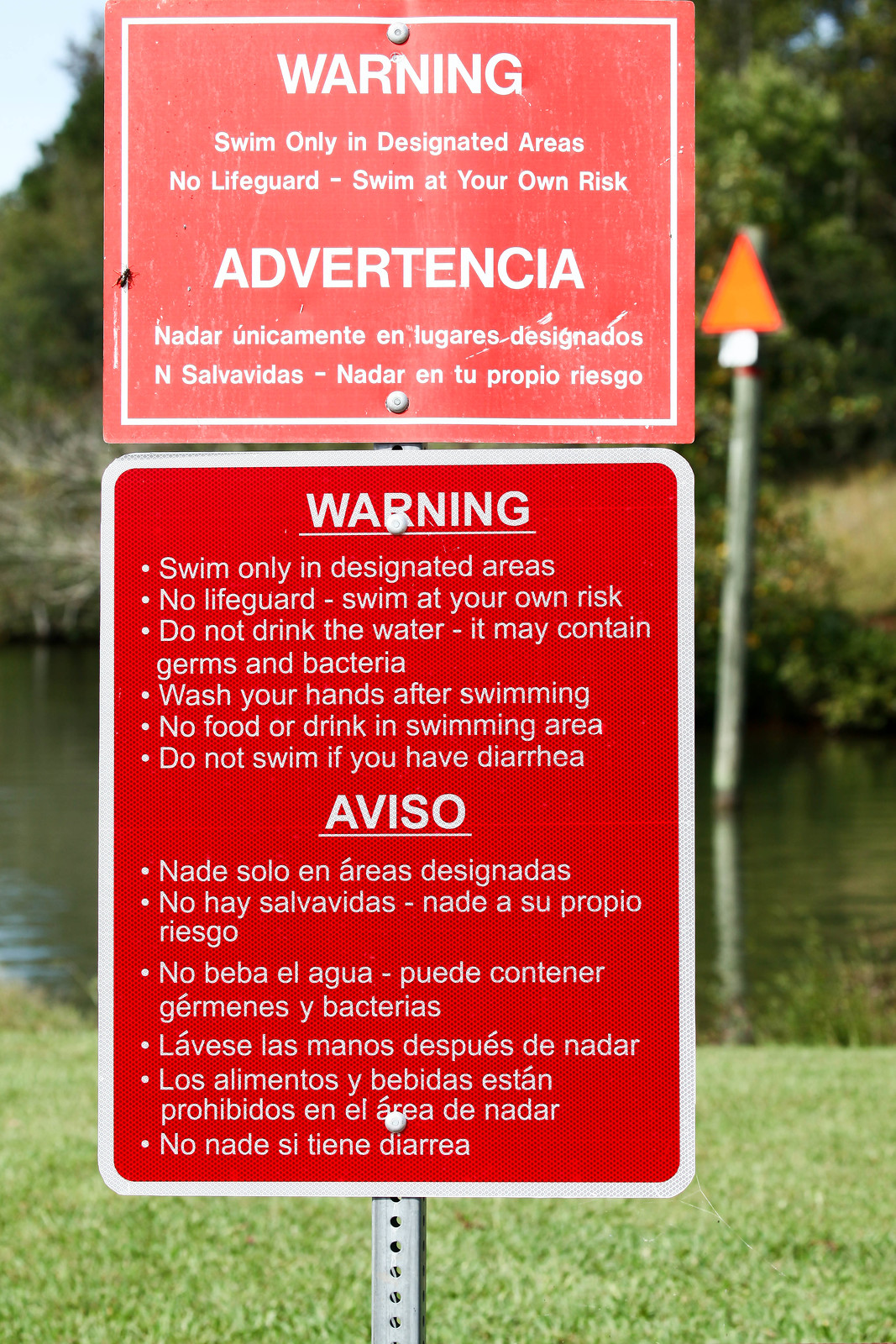The image depicts a pair of warning signs positioned by the edge of a red-hued body of water, likely a lake, surrounded by grass and trees visible in the blurred background. The top sign is light red with white text and a white border, stating: "Warning: Swim only in designated areas. No lifeguard, swim at your own risk," followed by the same message in Spanish: "Advertencia: Nadar únicamente en lugares designados. No hay salvavidas, nadar a su propio riesgo." Below this, a second sign in bright red with a white border and white text includes several bullet points. It reads: "Warning: Swim only in designated areas. No lifeguard, swim at your own risk. Do not drink the water, it may contain germs and bacteria. Wash your hands after swimming. No food or drink in swimming area. Do not swim if you have diarrhea," and is also translated into Spanish below: "Aviso: Nadar solo en áreas designadas. No hay salvavidas, nadar a su propio riesgo. No beba el agua, puede contener germenes y bacterias. Lave las manos después de nadar. Los alimentos y bebidas están prohibidos en el área de nadar. No nade si tiene diarrea." Both signs are mounted on a steel pole, ensuring they are securely fastened and visible.